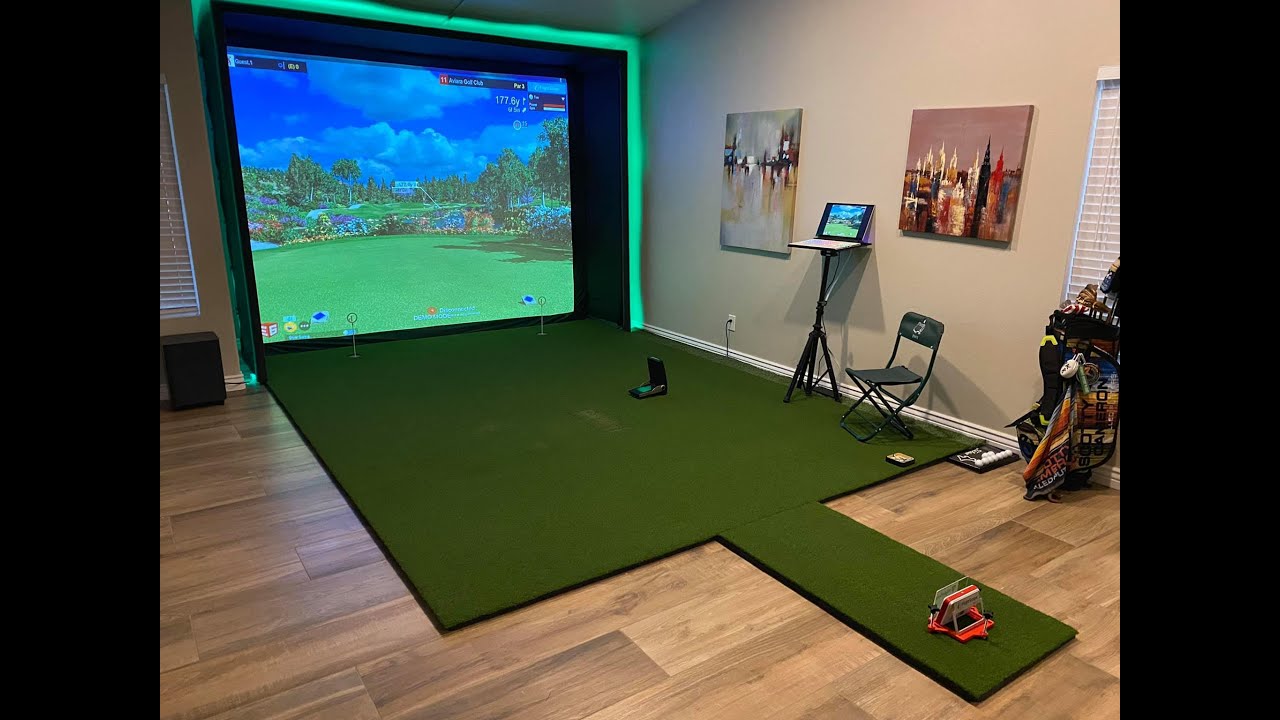This image depicts a dedicated golf simulator room within a house, featuring a large screen on the back wall that showcases a virtual golf course with realistic elements such as grass, flowers, trees, and a blue sky. This screen is outlined by an LED green border, enhancing its visual appeal. In front of the screen lies a square area of artificial turf where one can practice their golf swings. The rest of the floor is wooden, giving a warm contrast to the green turf. Positioned off to the side, a tripod stand supports a computer that likely controls the simulator program. Nearby, a golf bag filled with clubs is ready for use, and a small fold-out chair provides seating. The beige walls are adorned with two canvas wall arts—one horizontal and one vertical—contributing to the room's aesthetic. Additionally, there is a small window partially covered by a blanket. Overall, the room combines functional design with decorative details to create a sophisticated and immersive golfing environment.